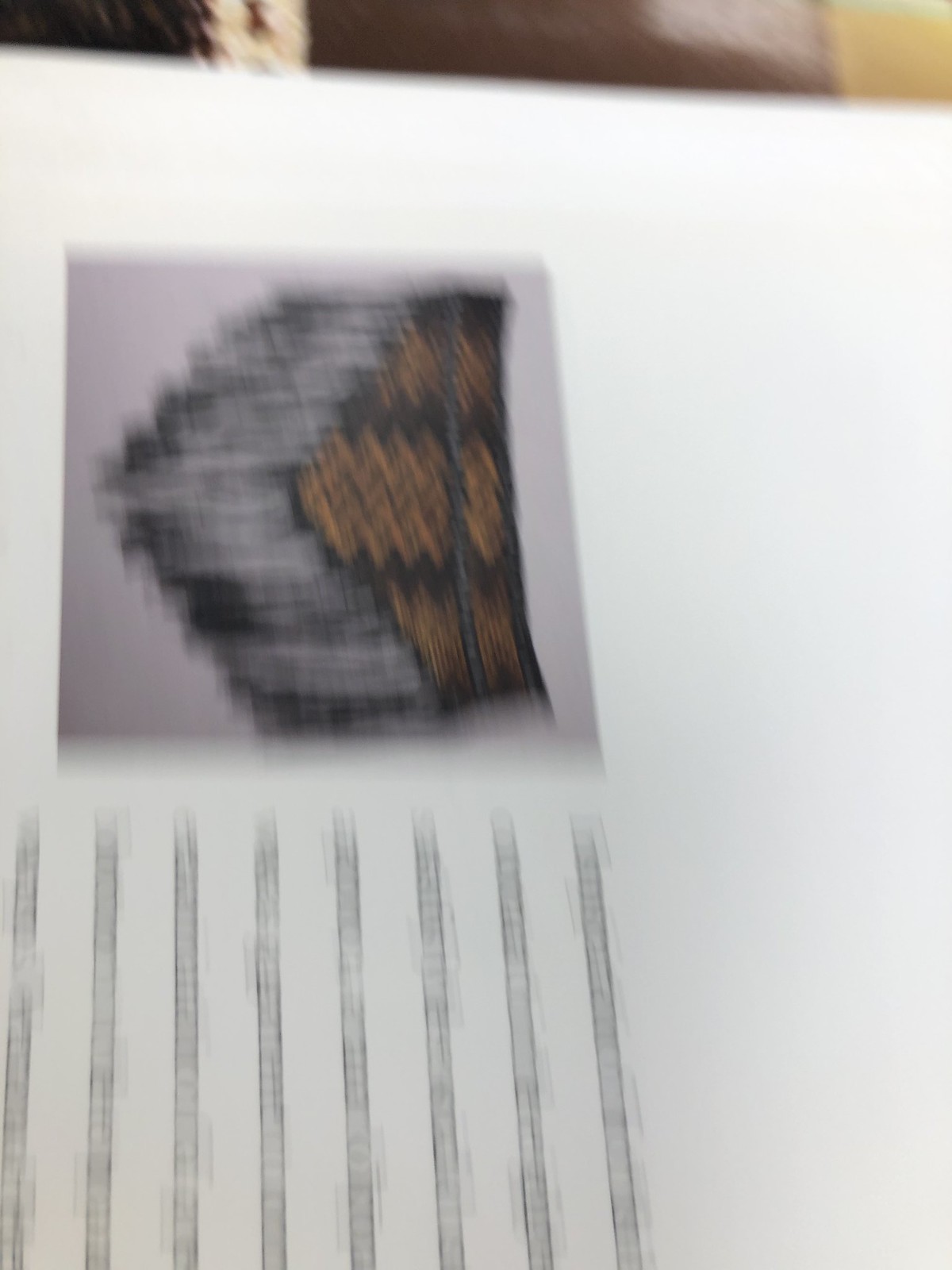This photograph, presented in portrait orientation, captures a rectangular sheet of white paper positioned sideways. At the upper section of the paper, there is a blurry image dominated by brown and gray hues. Beneath or adjacent to the image are several lines of indistinct text, which are challenging to decipher due to the blur. The backdrop visible at the top of the photo features a blend of brown, tan, and off-white shades.